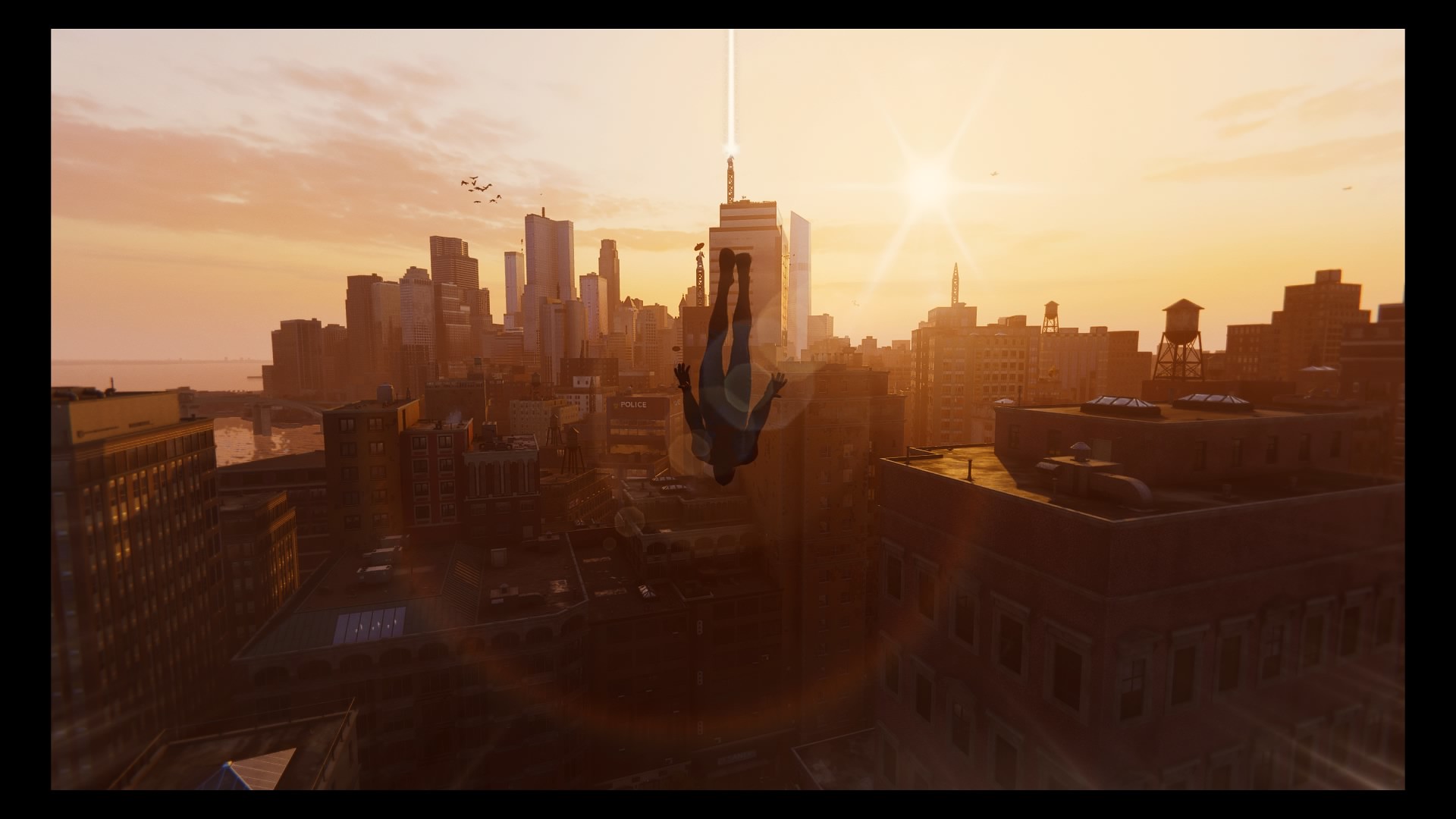This image appears to be a computer-generated or animated depiction of an urban landscape, most likely a large city akin to New York. The skyline features numerous skyscrapers, water towers, and a variety of residential buildings. There's a yellow-orange glow enveloping the scene, suggesting a sunset with a notably pinkish and low-lying cloudy sky. Birds are visible in the background, adding a natural element to the urban environment.

At the forefront of the image is a dark, shadowy silhouette of a male figure with elongated limbs, seemingly suspended in mid-air or falling headfirst, implying a superhero or paratrooper. This figure is accentuated by multiple rings of light, likely sunspots caused by the reflection of the setting sun. The bright sunlight casts a vivid glow over the entire scene, highlighting the cityscape in striking detail. Additionally, there is a hint of a distant body of water, possibly an ocean or a lake, with a solitary boat visible on its surface. The photo's border is marked by a dark perimeter, framing the graphic design or illustration.